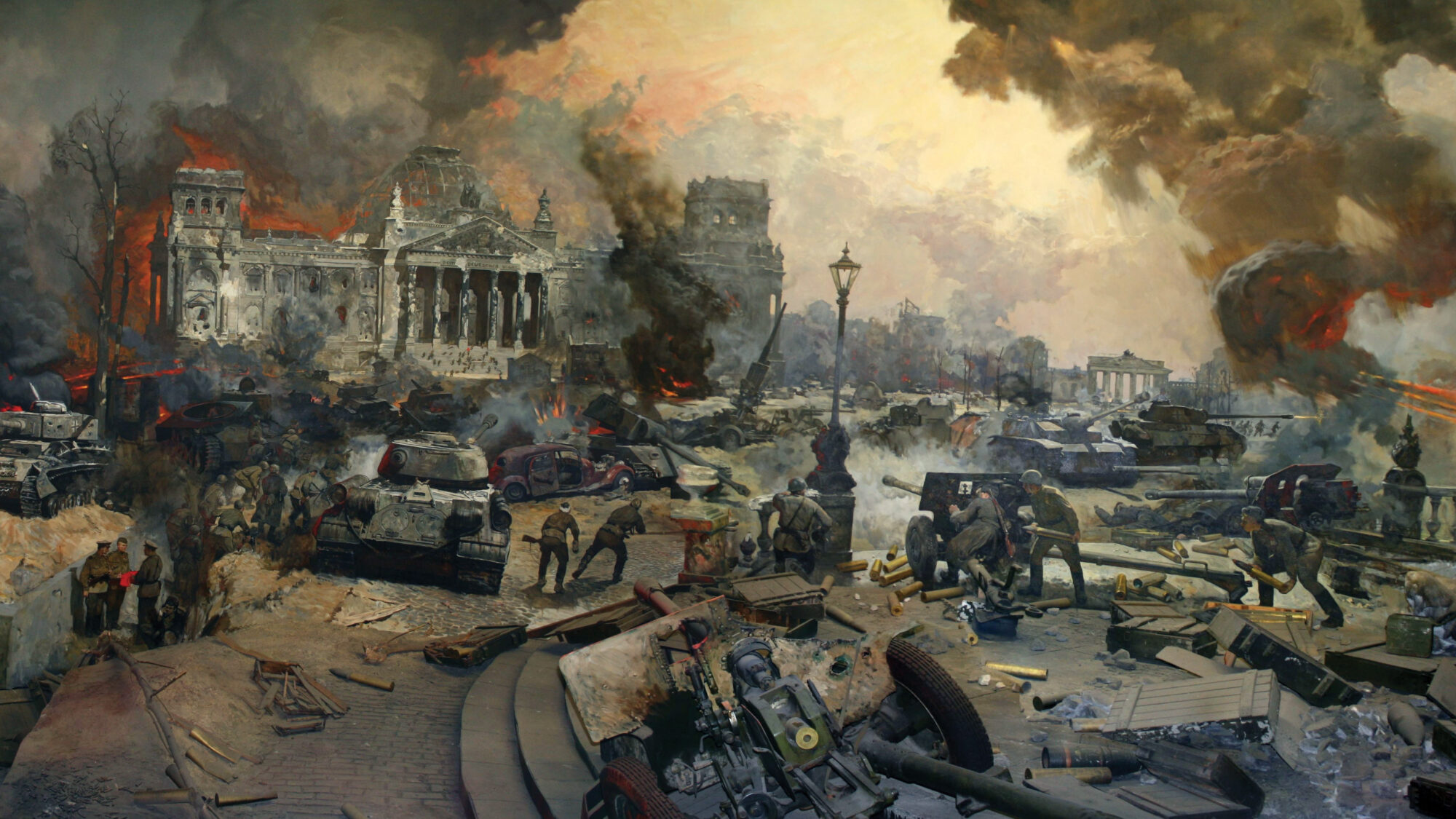The image depicts a chaotic war zone, captured in an oil painting style, likely representing an old-fashioned city engulfed in flames and smoke. Predominantly rendered in grays, the scene is colored with the vivid reds and oranges of the fire. The background features a large, classical white building ablaze, with gray smoke billowing from it, standing prominently to the left. The sky above is dominated by dark black, gray, and brown smoke, interspersed with patches of red and orange flames, creating a foreboding atmosphere. 

The foreground is densely populated with soldiers clad in uniforms and helmets, armed and actively engaged in combat. Some soldiers are seen loading missiles into cannon-like guns, adding to the air of intense conflict. Amidst the chaos, several gray tanks are strategically placed, and behind makeshift shields, men operate gun emplacements. To the lower left, three uniformed officers, distinguishable by their red scarves, seem to be in a discussion, perhaps strategizing amidst the disorder. The right portion of the image is marked by a significant puff of orange fire combined with black smoke, while scattered equipment and what looks like snow cover parts of the ground, accentuating the scene's devastation. The remnants and the depicted actions underscore the catastrophic aftermath of a brutal battle.